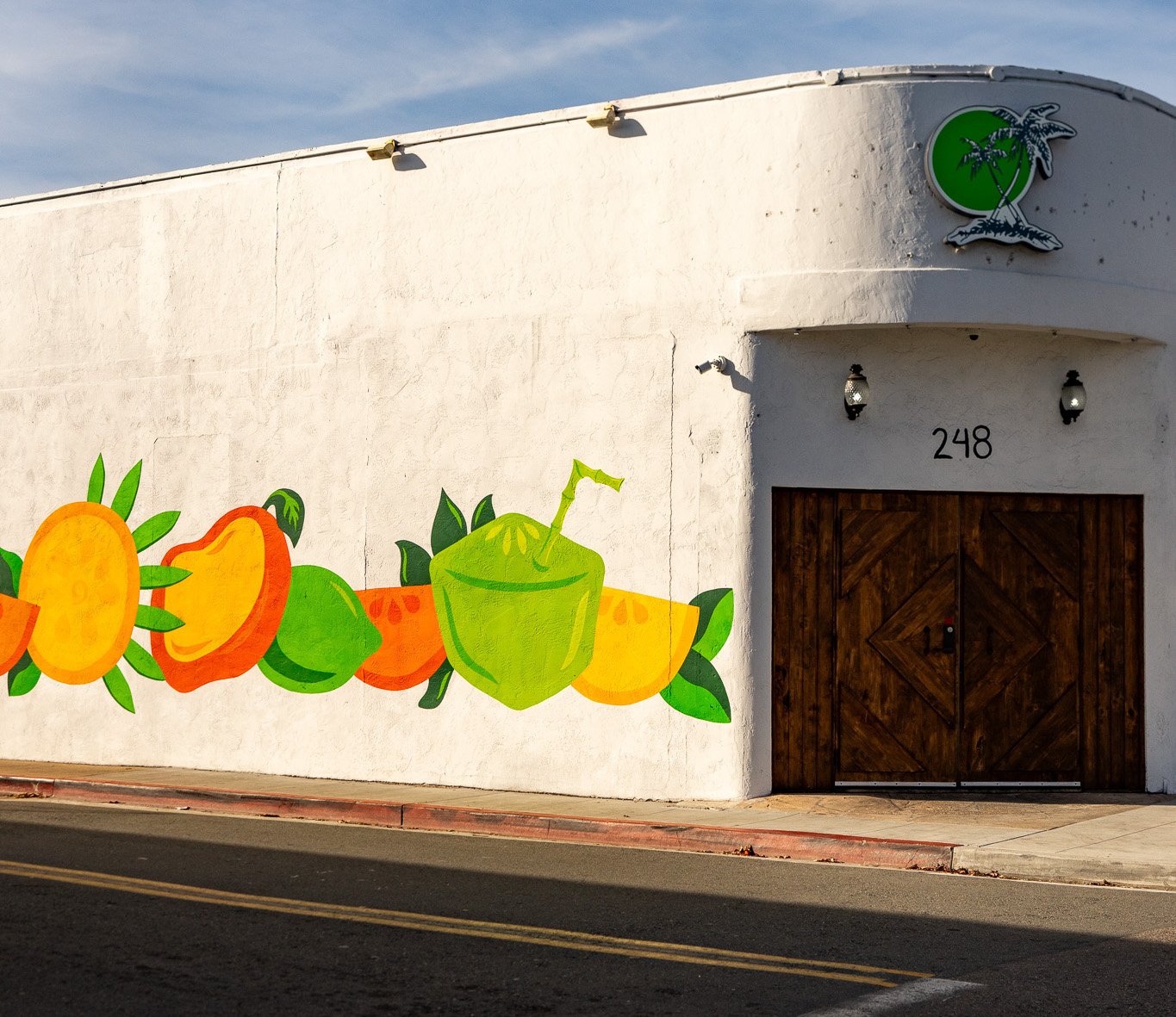Captured in a landscape-oriented color photograph, this image reveals a short, flat-roofed building at the corner of an intersection. The white stucco exterior features a curved corner where the main entrance is located, marked by the number "248." This entrance, comprised of dark wooden double doors, is highlighted by twin light fixtures above. Over the doorway, a striking neon sign portrays a green circle adorned with palm trees. Adorning the side wall of the building is a vivid mural in a photographic representational realism style, displaying a colorful array of fruits and vegetables. The mural includes elements such as apple slices, lime, orange, lemon peels, watermelon, and spinach, laid out in a visually appealing horizontal format. The scene is set under a bright blue sky with white misty clouds, suggesting a sunny day, and the gray asphalt road in the foreground contrasts with the vibrant colors of the mural.